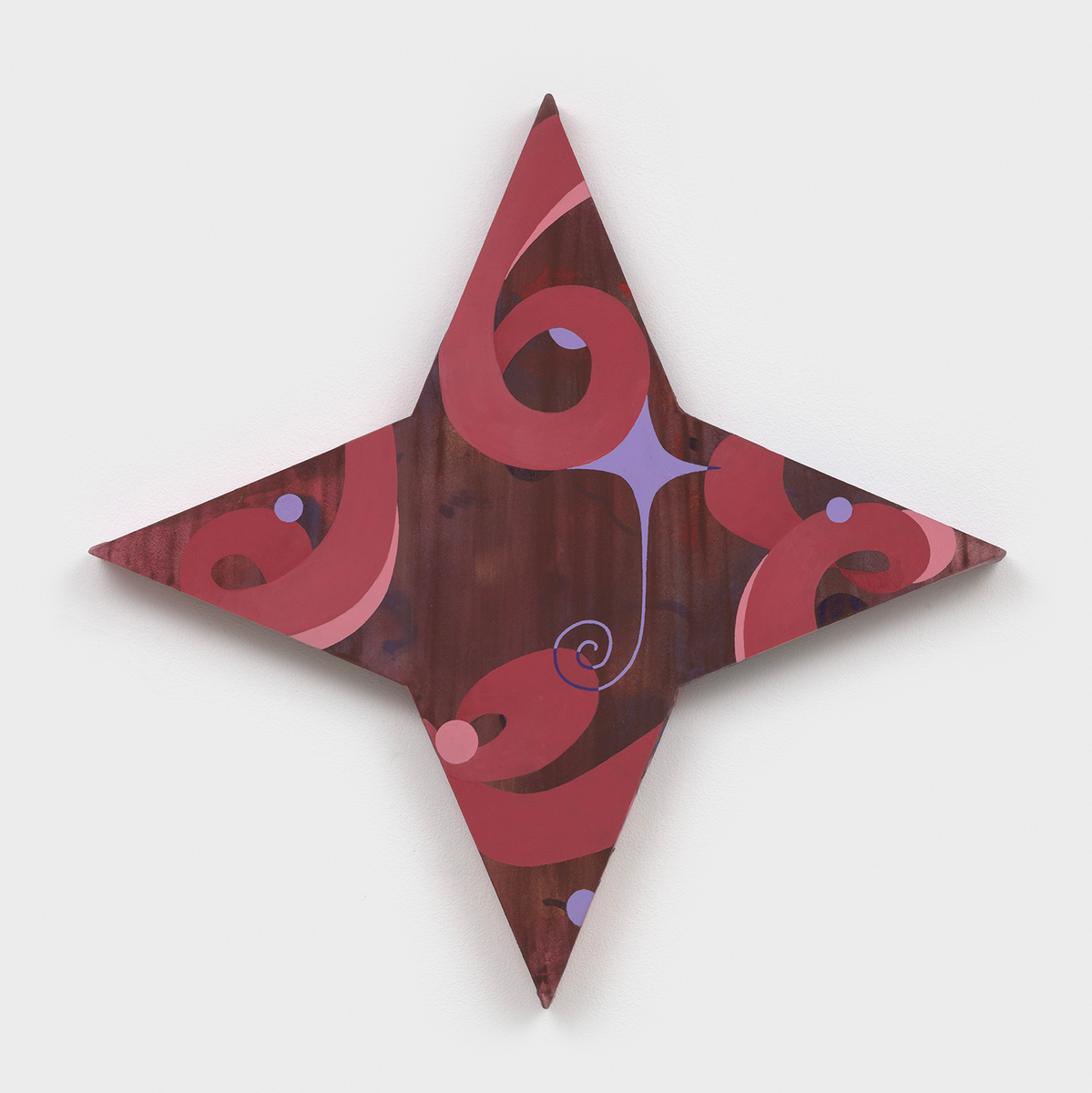The image features a central four-pointed star that conveys a three-dimensional effect, thanks to a drop shadow giving it depth. The surface behind the star is an off-white color with a subtle wood-grain texture, casting shadows in two directions, which adds to its dimensionality. The star has a brownish hue and is framed by an intricate design of accented swirls and polka dots. Each corner of the star is adorned with red swirls: the top one resembling a red number six, the left and right points featuring slightly different red swirls, and the bottom one looking like a sideways six. Additional embellishments include a purple swirly shape dripping from the top swirl, and randomly placed polka dots in various sizes, predominantly purple and pink. The entire composition achieves an artsy, craft-like aesthetic with the swirls and dots providing a dynamic, playful element to the design.